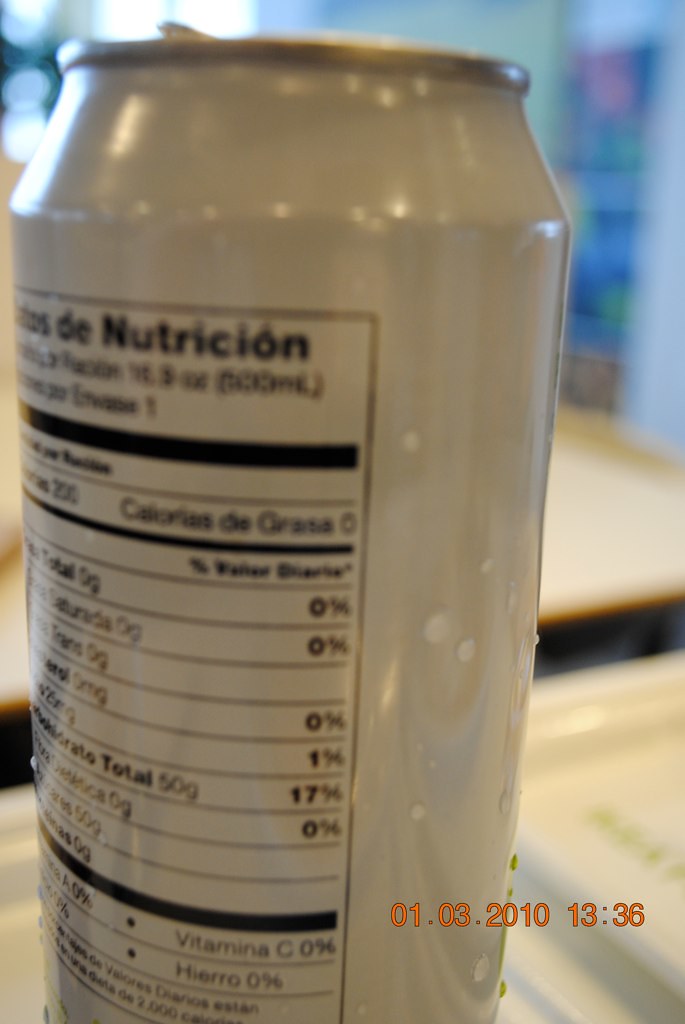This real-life close-up photo features a white aluminum soda can, set against a blurry interior backdrop that suggests it's on a shiny countertop, possibly in a restaurant. The can is angled, showing half of a Spanish nutrition label, partially readable with details such as "200 calories," "calories de grasa: 0," "total fat: 0g," "saturated fat: 0g," "trans fat: 0g," and "cholesterol: 0mg." Other nutritional information includes "carbohydrates: 50g (17%)," "potassium: 0g," "Vitamin A: 0%," "Hierro (Iron): 0%," and "Vitamina C: 0%." The image quality is low, possibly due to poor focus or a low-resolution camera, but the can's minimalistic design can be discerned, with "de nutricion" in black text on a white background. Additional elements include a blue blurry rectangle on the wall, possibly a menu, and tan tables, hinting at a restaurant setting. The bottom right corner of the image is timestamped in orange with a black outline: "01.03.2010 13:36."